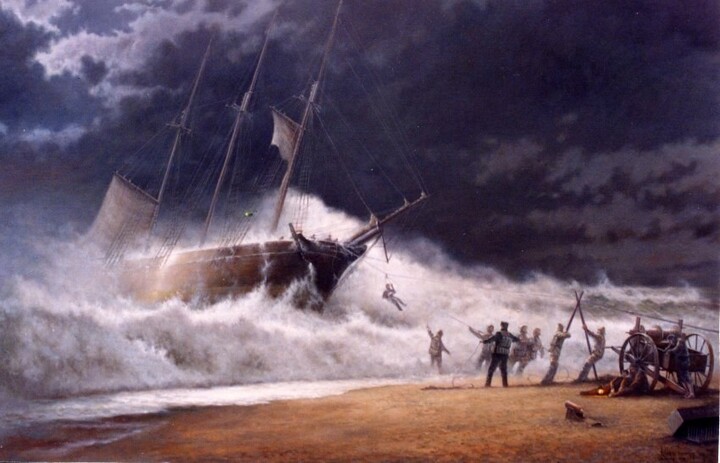The painting depicts a dramatic scene of a shipwreck at the beach. A large brown ship with white sails, torn and battered, struggles against massive, choppy waves that are crashing onto the shore. Amidst the tumultuous sea, a man is seen zip-lining down a pulley line from the ship towards safety. On the sandy shore, partially in shadow from the dark blue sky dotted with ominous white and gray clouds, a group of men is gathered. They are intently maneuvering a two-wheeled apparatus, which appears to be part of a rescue effort. One man is waving, while others seem to be erecting a pole for the zip line. Interestingly, there's a cannon on the shore, likely salvaged from the distressed ship. The scene exudes tension and urgency, capturing the perilous endeavor to rescue the ship's crew from the stormy seas.